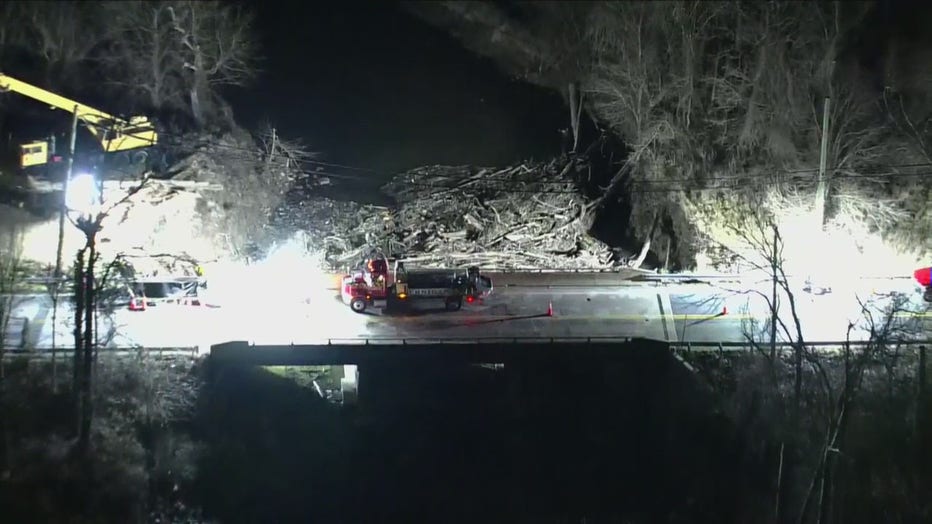In this detailed nighttime scene, a large-scale operation is illuminated by giant spotlights on a bridge. The image captures a bustling worksite where a red tow truck equipped with a black trailer and an articulating arm is attempting to clear a massive log jam beneath the bridge, likely caused by a recent flood. The arm of the truck is visibly reaching down into the debris, working tirelessly to restore the water flow. Surrounding the truck are numerous hazard cones positioned to control traffic and ensure safety. Additionally, perched nearby is an earth mover, a heavy yellow truck with a large extension, indicating extensive excavating work. The bridge spans over water, which is dark and difficult to see clearly, and the area below the bridge is shrouded in darkness. The surrounding environment, consisting of leafless trees, suggests a winter setting without any snow. The scene is further accentuated by the stark, bright lights contrasting against the dark night, highlighting the urgency and intensity of the ongoing project.